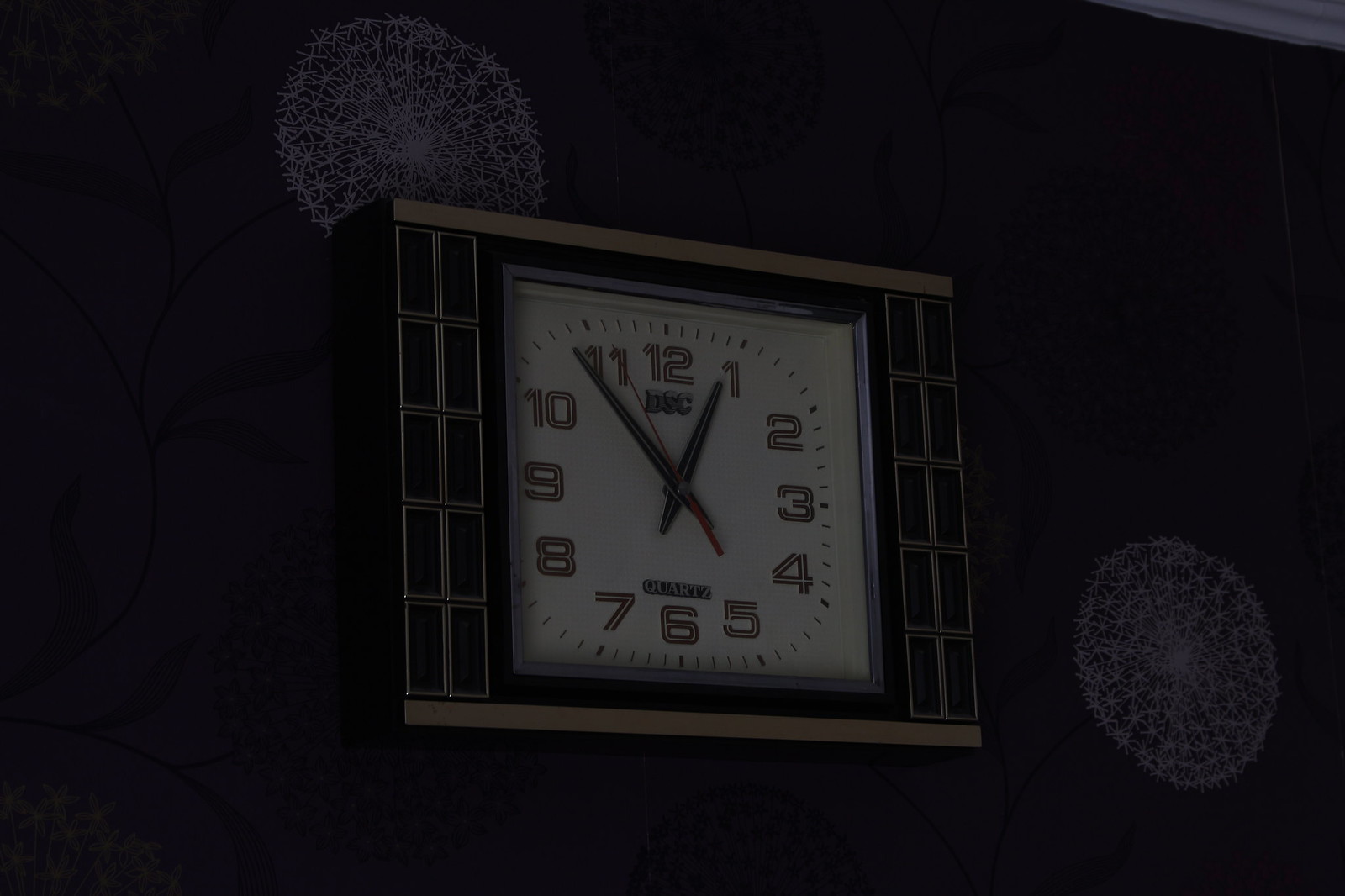This image showcases a wall-mounted clock set against a wallpapered background. The wallpaper features a deep blue-purple hue adorned with an intricate pattern of vines interspersed with white, dandelion-like designs. The clock itself is square-shaped with distinct black borders on either side, accentuated by gold horizontal bars at the top and bottom. The clock face prominently displays the brand "DSC" just beneath the number 12, adding a touch of elegance to its overall design.